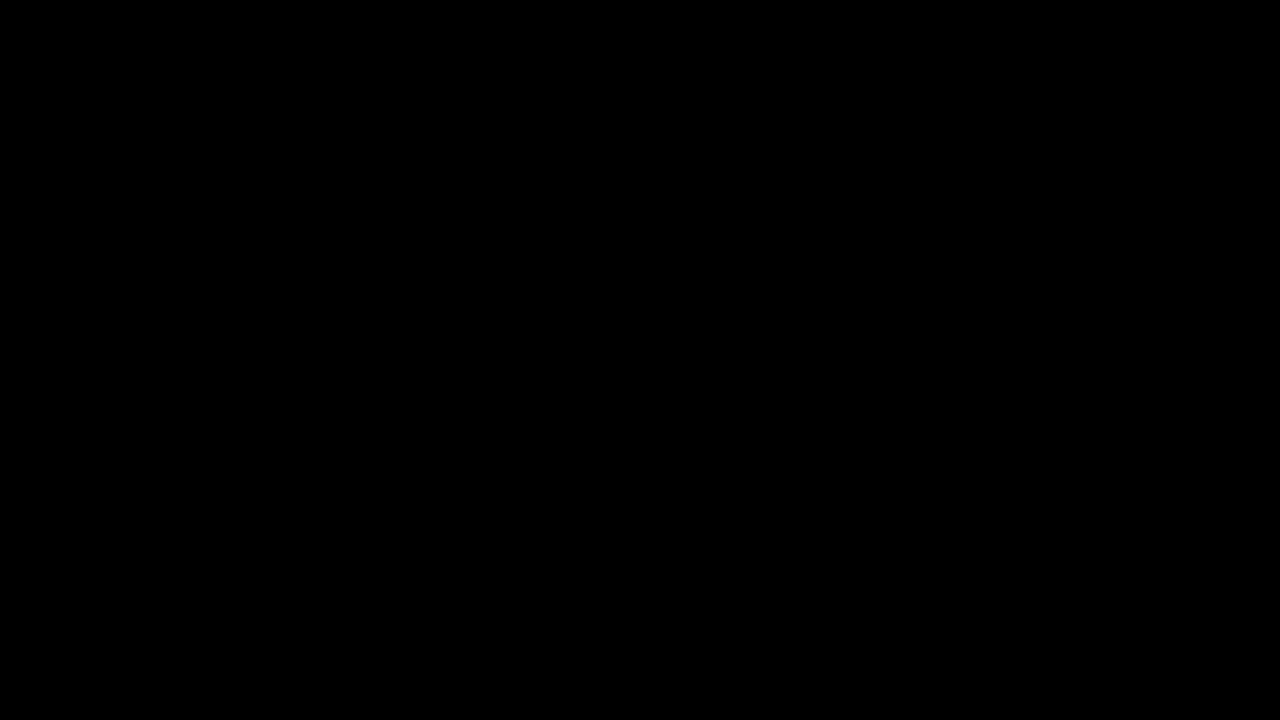This image features an entirely solid black rectangle, devoid of any text, design, or objects. The rectangle is pitch black, creating a void of color where no shading or variations are present. The shape is precisely rectangular with sharp, well-defined corners, oriented horizontally so that it is longer from left to right than it is in height. The image is void of anything else, embodying simplicity with its pure midnight black hue dominating the entirety of the space.